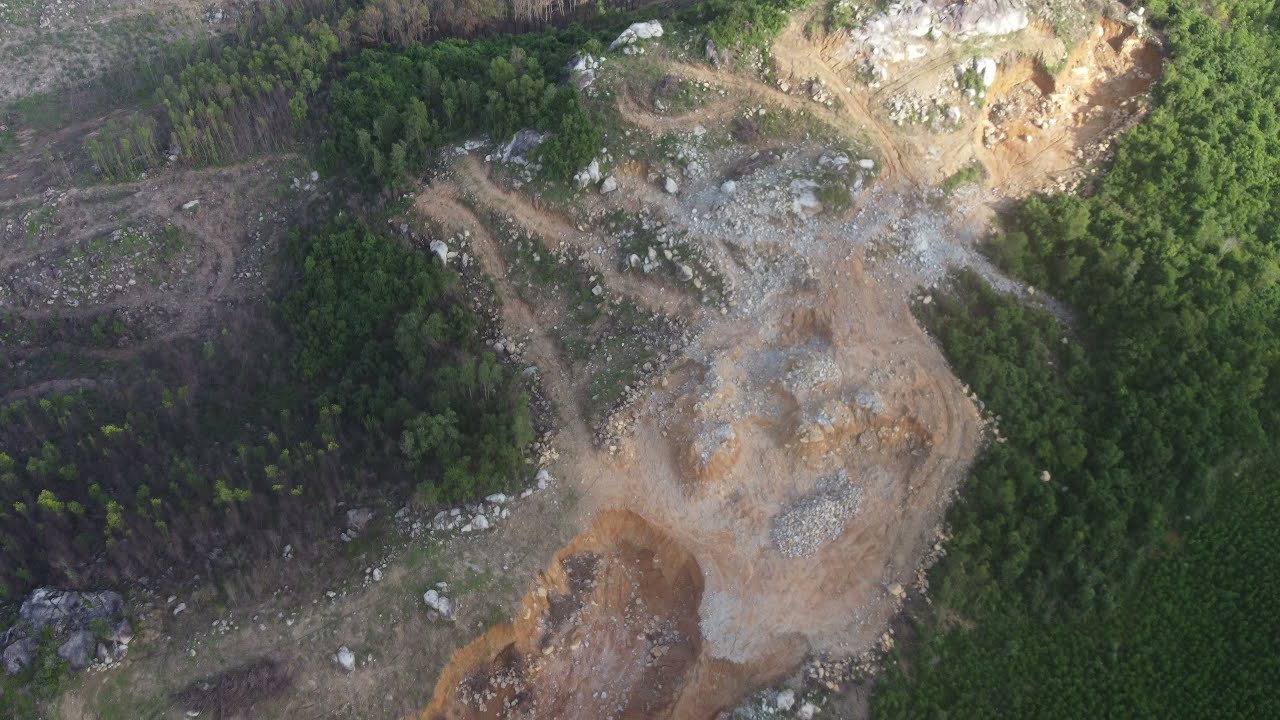The aerial photograph, likely taken by a drone from about 100 feet above ground, captures a sunlit and shaded rocky landscape. In the center of the image is a large, uneven brown dirt mound peppered with several large, white rocks and scattered green plants. This appears to be a dirt biking area, complete with multiple dirt paths crisscrossing through it. Dense green vegetation and trees surround the dirt patch, with small paths weaving in between the foliage. The upper right portion of the image is brightened by sunlight, while the rest remains under a shadow, possibly due to clouds or mountain terrain. The lower right corner features a dense forest, contributing to the overall lush greenery that frames the rocky centerpiece.